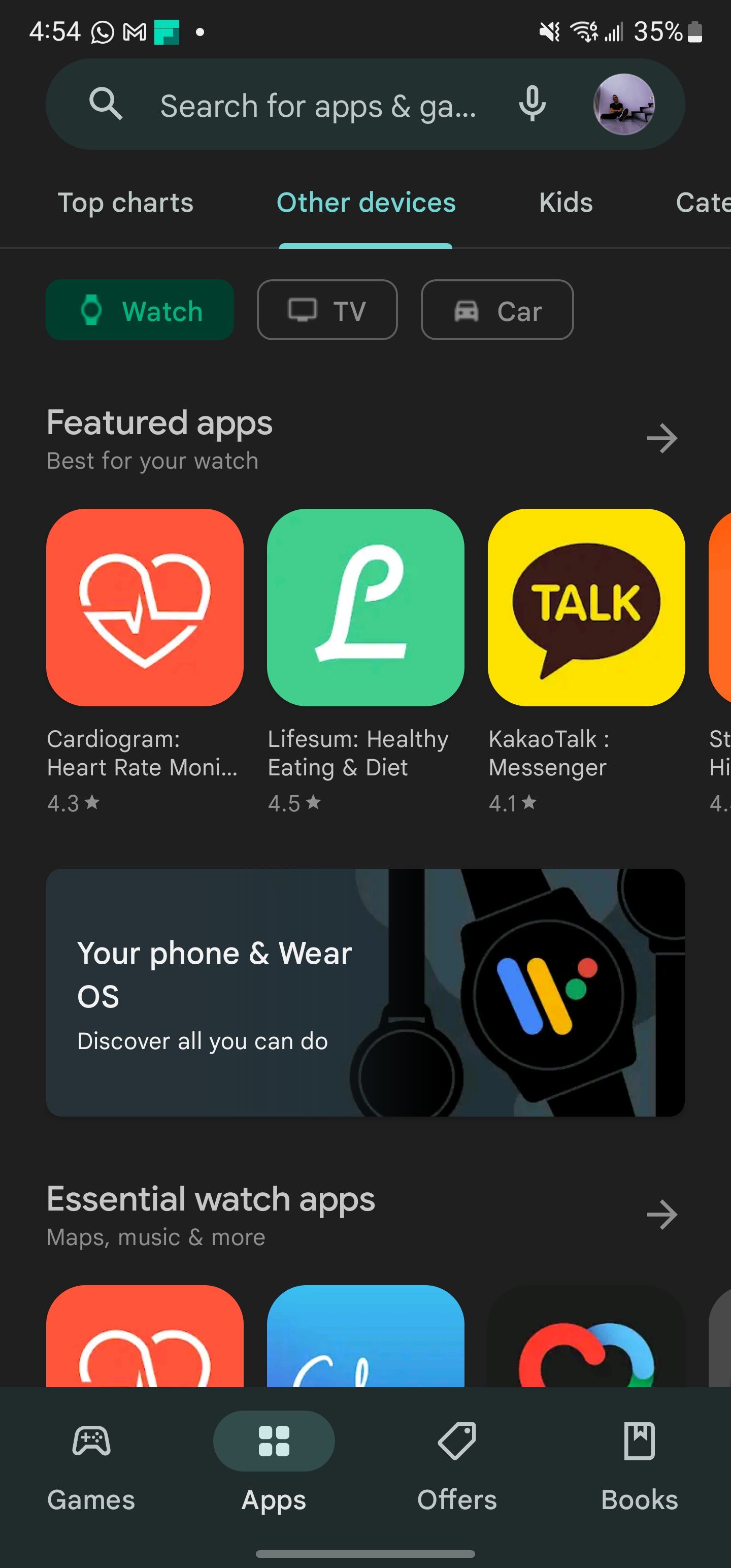The screenshot captures a mobile phone screen displaying the Google Store app. In the upper left-hand corner, the time is shown as 4:54 alongside an 'M' icon indicating a new Gmail message. Other status icons display a battery life of 35%. At the very top, there's a search bar in the form of an oval.

The screen is displaying the section for "Top Charts" under the category of different devices, specifically focusing on "Kids." There are buttons for various devices including watches, TVs, and cars, with a prominent button labeled "Watch" to indicate featured content for smartwatches.

A highlighted section lists "Best for Your Watch," featuring apps such as Cardiogram, Lifesum for healthy eating and diet, and a talk messenger. Following this, the page outlines sections dedicated to "Your Phone" and "Wear OS" with images of watch faces, promoting the discovery of various features.

Further down, it points to "Essential Watch Apps" that include Maps, Music, and more. At the bottom of the screenshot, there are navigation icons for Games, Apps, Offers, and Books, providing easy access to other sections of the Google Store.